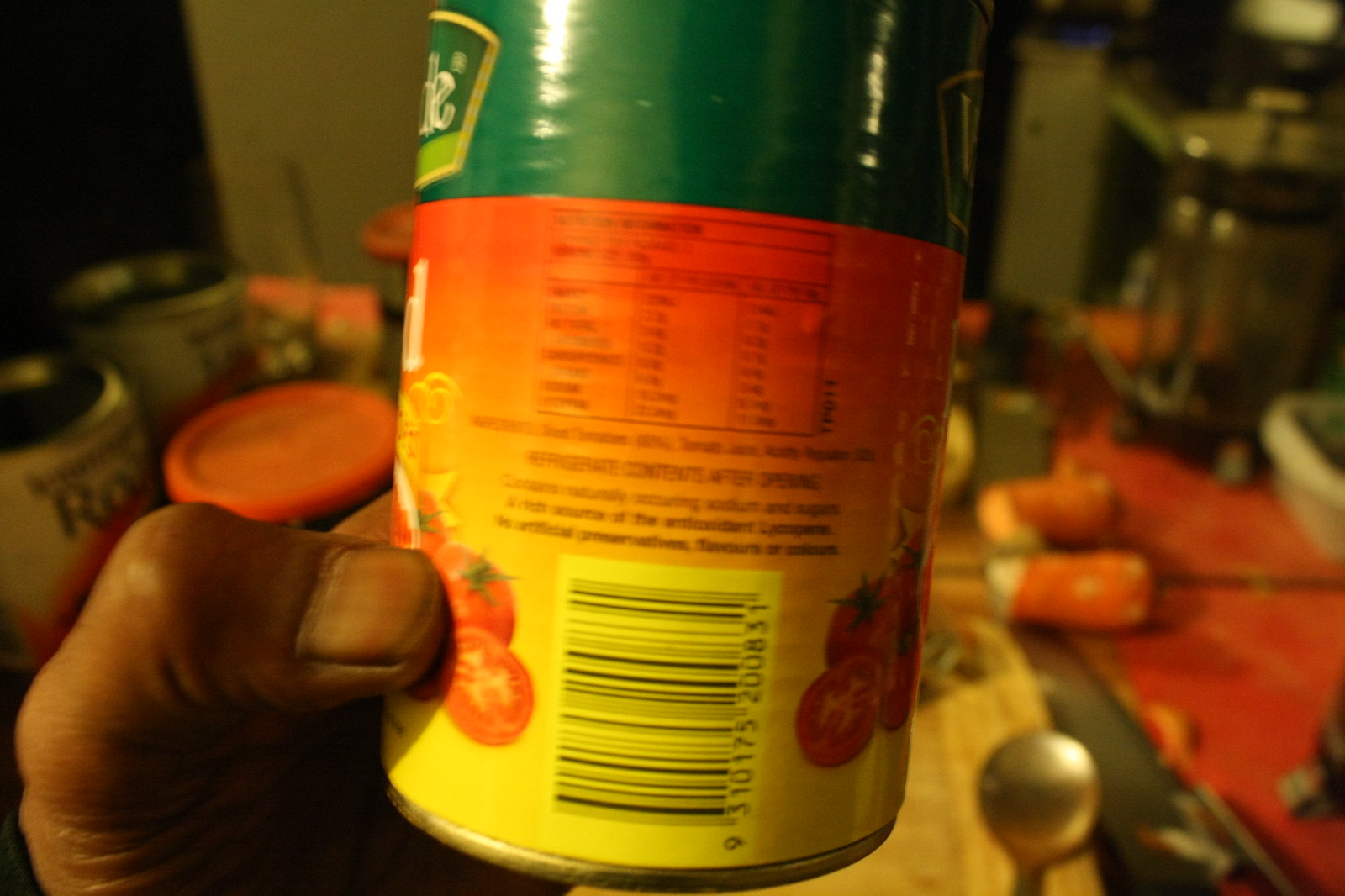The image portrays a canned food product being held by a left hand, with a visibly dirty thumbnail, likely belonging to a black person. The can's design features a top section with a green background, extending horizontally across the entire can, adorned with a partially visible logo on both the left and right sides. Below the green band, the can transitions into a red and yellow gradient background. 

At the very top of this section rests a nutrition facts chart accompanied by an ingredients list, though the text is unreadable due to the image's blurriness. The can's bottom portion includes a prominently displayed barcode, flanked by images of tomatoes—some of which are shown sliced. Below the barcode, the numbers "9310175207831" are discernible. Just above this, there is a black text advising to refrigerate the contents after opening.

The background of the image reveals a kitchen setting with a wooden cutting board positioned centrally, supporting a silver spoon. To the right, a French press is visible, alongside two more cans to the left. The entire image appears notably blurry and out of focus, obscuring finer details and making some text challenging to read.